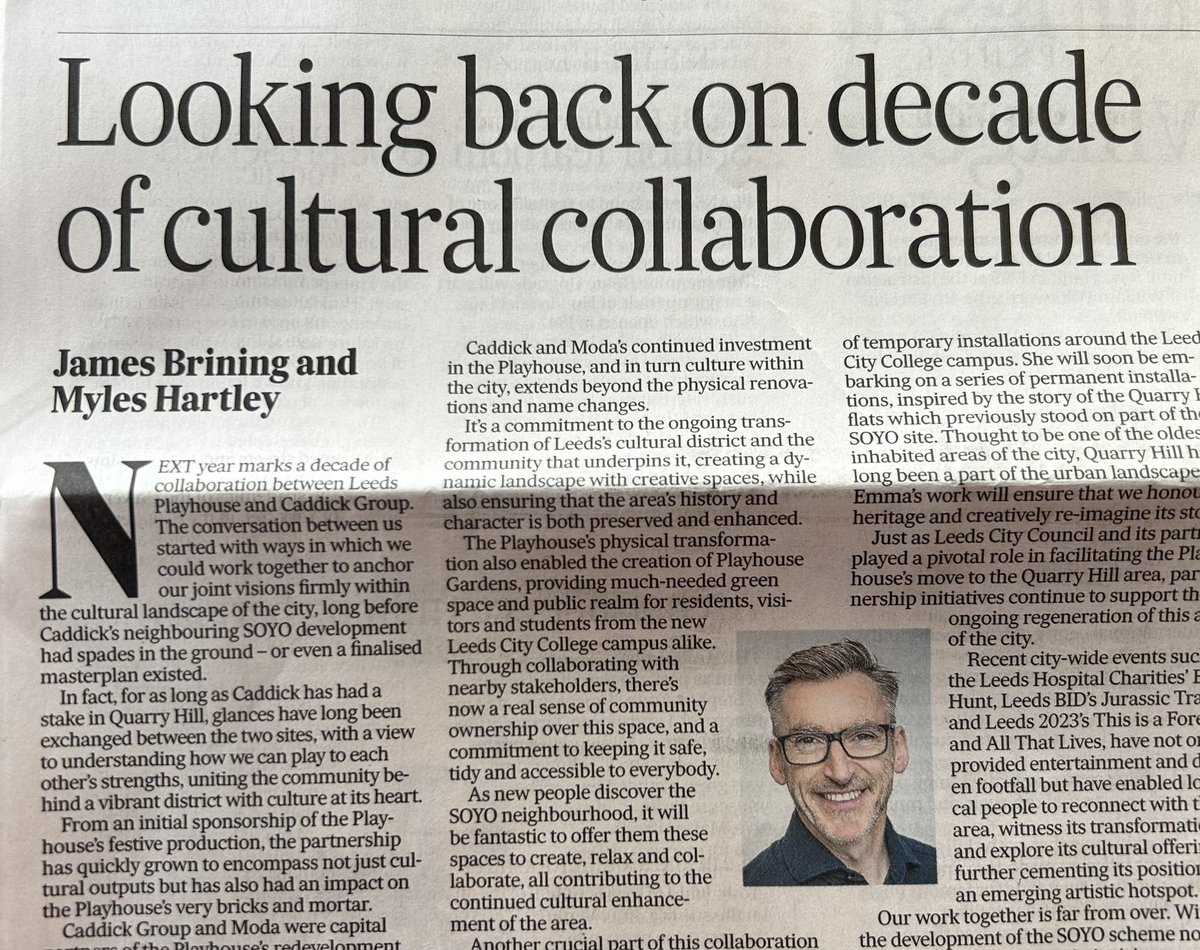This photograph captures a newspaper clipping featuring a prominently folded crease running horizontally across the middle, obscuring portions of the text. The clipping's first two paragraphs are fully legible, while the second column contains four readable paragraphs. However, the third column's text is truncated on the right side due to the fold. Positioned between the second and third columns, a photograph of a man is displayed. This man has a mix of gray and brown hair, styled back from his forehead, and sports black-framed glasses. He's smiling, revealing his top row of teeth, and has a bit of stubble. He is dressed in a blue shirt. The headline of the article reads "Looking Back on a Decade of Cultural Collaboration," penned by James Brinning and Miles Hartley. The introductory word of the article begins with an embellished capital "N," and the text commences with: "Next year marks a decade of collaboration between Leeds Playhouse and Caddick Group."